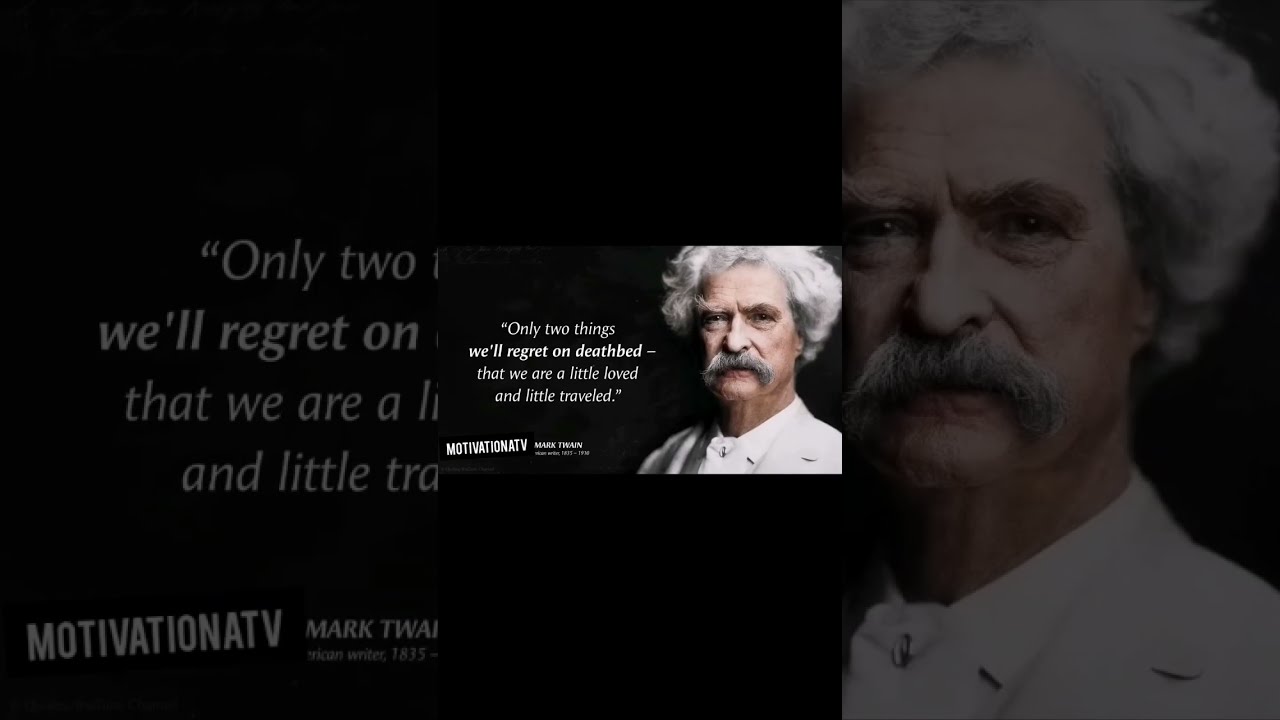This image features a sophisticated, AI-generated portrayal of Mark Twain on the right, characterized by his fluffy white-gray hair, bushy eyebrows, and mustache. His seasoned face, marked with lines and wrinkles, captures a neutral expression as he looks straight at the camera, donning a white shirt and jacket against a splotchy, dark background. On the left side of the image is one of Twain's poignant quotes, written in a rectangular caption: "Only two things will regret on deathbed, that we are little loved and little traveled." The quote stands prominently, reinforcing the theme of life's fleeting nature. At the bottom left corner, the editor's credit, "Motivation ATV," is distinctly displayed. This composite image is minimalist in design, with the central focused content set against a holographic duplication of the same image in the background, creating a layered effect.